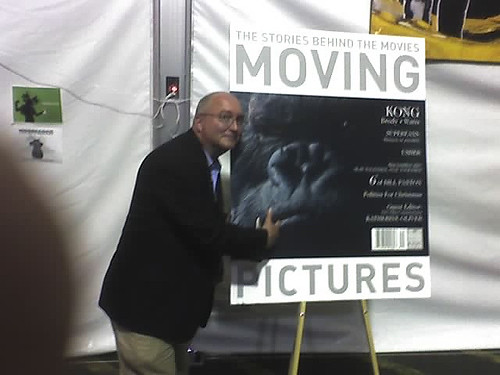In the image, a man who appears to be in his late forties, with balding gray hair and glasses, stands on a stage beside a large rectangular poster mounted on an easel. The man is dressed in a black suit jacket, a light blue button-up shirt, and light tan khaki pants, and he appears to be presenting the poster, possibly at a convention or a book signing. He is leaning forward and pointing at the poster with a smile. The poster, designed to resemble a book cover, prominently features a large, zoomed-in photograph of a gorilla, suggesting it is a depiction of King Kong. The top and bottom portions of the poster have white bars, with the top bar containing the text "The Stories Behind the Movies" and the word "Moving" in bold gray letters. Below the gorilla image, the bottom bar reads "Pictures" in similarly bold letters, forming the full title "Moving Pictures." Although other elements of the text on the poster are blurred and difficult to read, the overall presentation suggests the man could be the author of the book or a speaker discussing the content featured on the poster.